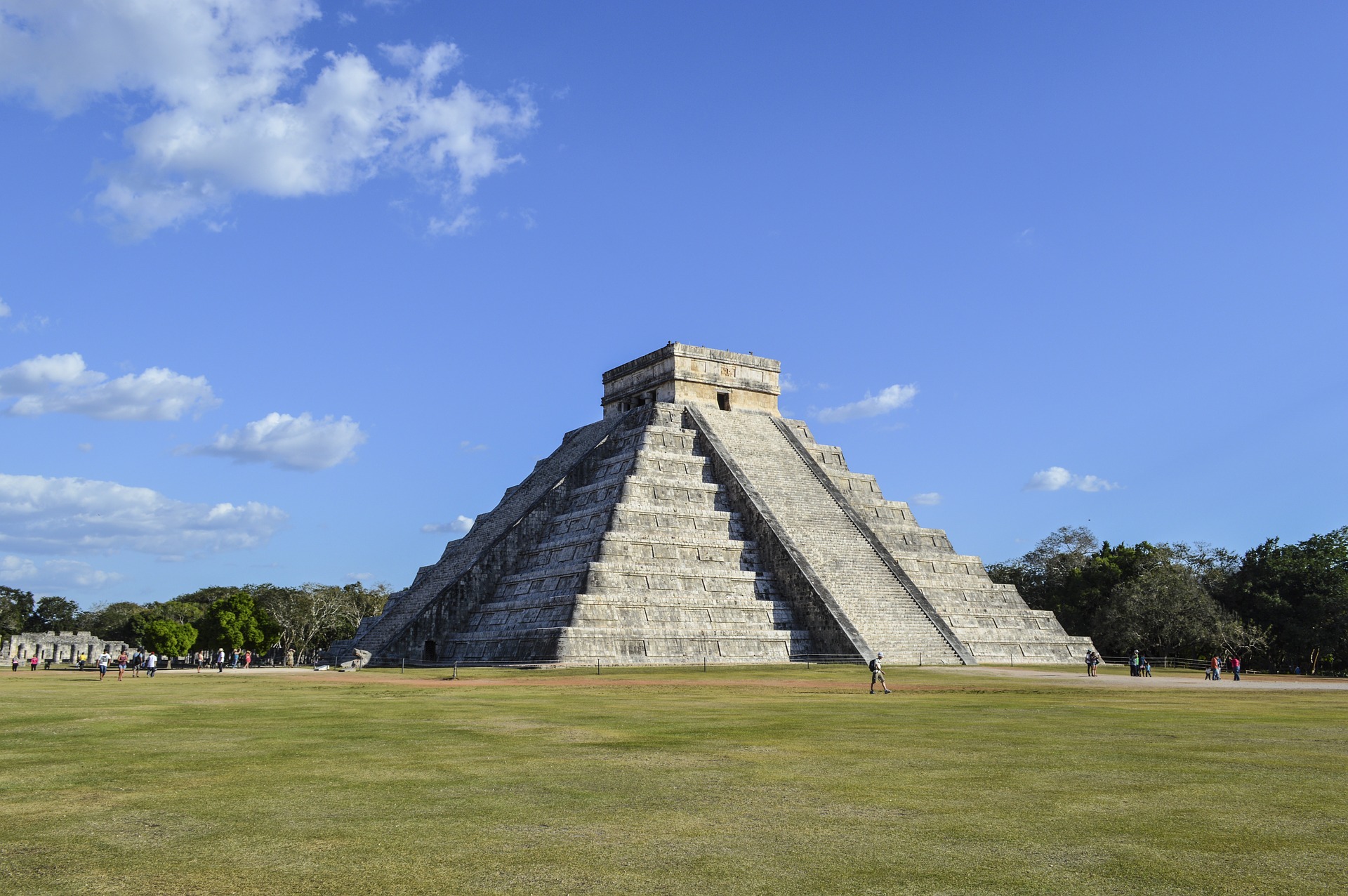The image depicts the majestic Chichen Itza pyramid in Mexico, prominently set against a brilliant blue sky scattered with a few wispy clouds. The stone structure, built from gray-white rocks, stands tall with approximately nine or ten levels, each resembling a series of step-like structures leading up to a small, square top. The pyramid features notable flat, slide-like rock ramps on the front and left side, which intrigue with their formidable stone construction. Surrounding the pyramid is a lush green landscape, with vibrant grass in the foreground and verdant trees in the background. Tiny figures of people can be seen mingling around the pyramid, both on the left and right sides, adding a sense of scale to the massive structure. Additionally, a white building can be spotted in the left background, further contextualizing the scene within its historical and cultural setting.